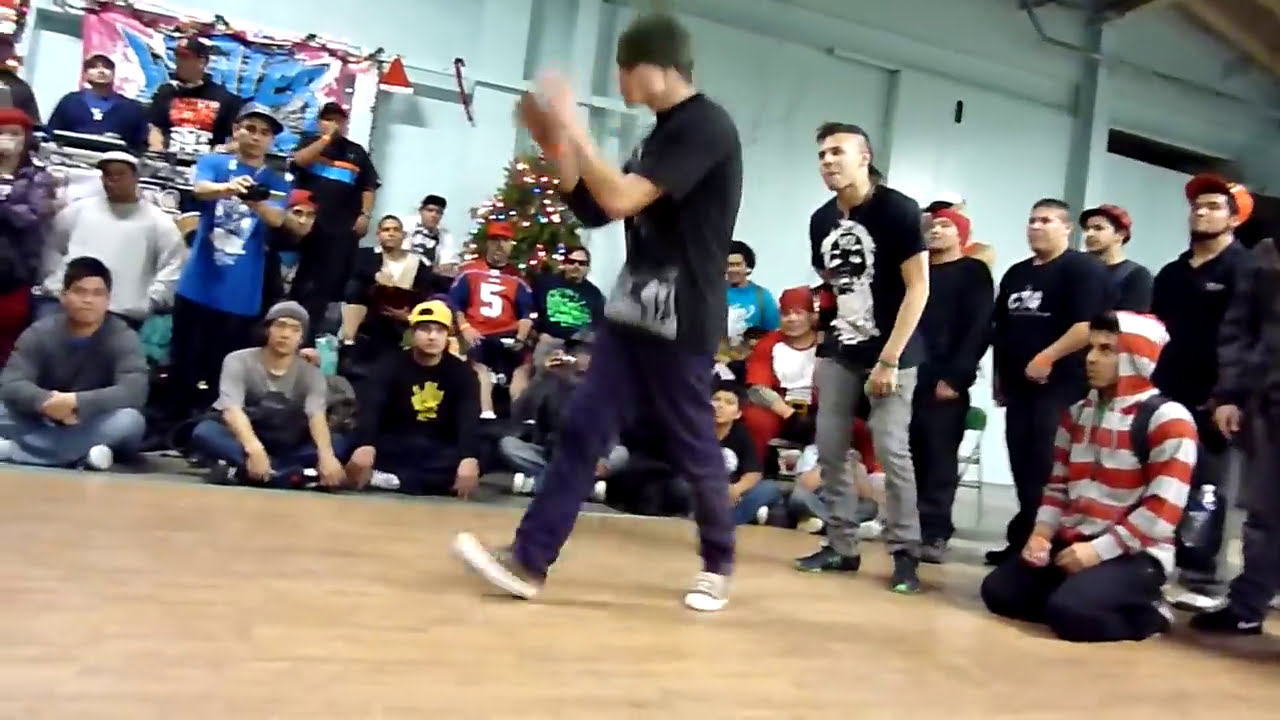The image captures a bustling interior space, resembling a gymnasium with its expansive wooden floor. At least over 20 casually dressed individuals, mostly with light-colored skin and dark hair, are either standing or seated around the room. The room’s walls are painted a light blue, and a Christmas tree is visible in the far background, adding a festive touch to the scene.

Dominating the center of the room is a man in motion, making him appear slightly blurred compared to the others. He's wearing a green beanie pulled low over his eyes, a black shirt, blue or possibly purple pants, and thin shoes reminiscent of Converse sneakers. His facial features are indistinct, either blurred out or seeming digitally altered. With his arms raised and partially together, he looks like he's about to clap or is mid-gesture.

Around him, people are arranged in a semi-circle, some standing, others sitting cross-legged or kneeling. Notably, one person on the far right is kneeling and wearing a distinctive red and white striped hoodie, black pants, and a backpack. Another individual to their left stands in a black shirt and gray pants. There's also a person with a blue t-shirt and black pants actively recording the central figure, suggesting an event or performance is taking place.

The detailed composition of the room, the described actions, and the attire of individuals contribute to an overall sense of a lively and engaged gathering in an informal, festive setting.